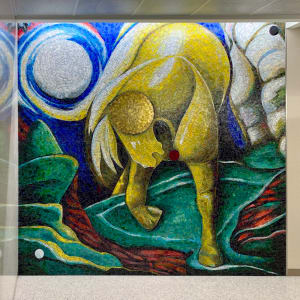The image is a vibrant and emotionally expressive piece of abstract art, likely a painting or mural. At its center, a prominently featured yellow figure, resembling a horse, stands out with its head inclined downward as if bowing or drinking from a shallow blue stream it appears to be walking through. The horse is detailed with yellow legs, hooves, and a white mane, adding to the intricate depiction. The background bursts with a dynamic palette of colors, including green, blue, white, and red, creating a variety of abstract shapes and patterns. In the top left corner, a large white circular shape reminiscent of the moon or another celestial body illuminates the scene. To the upper right, grayish stones or perhaps a cliff wall add texture and further complexity to the setting. The entire composition is bordered by a light gray frame, contributing to the structured yet expressive atmosphere of the artwork.